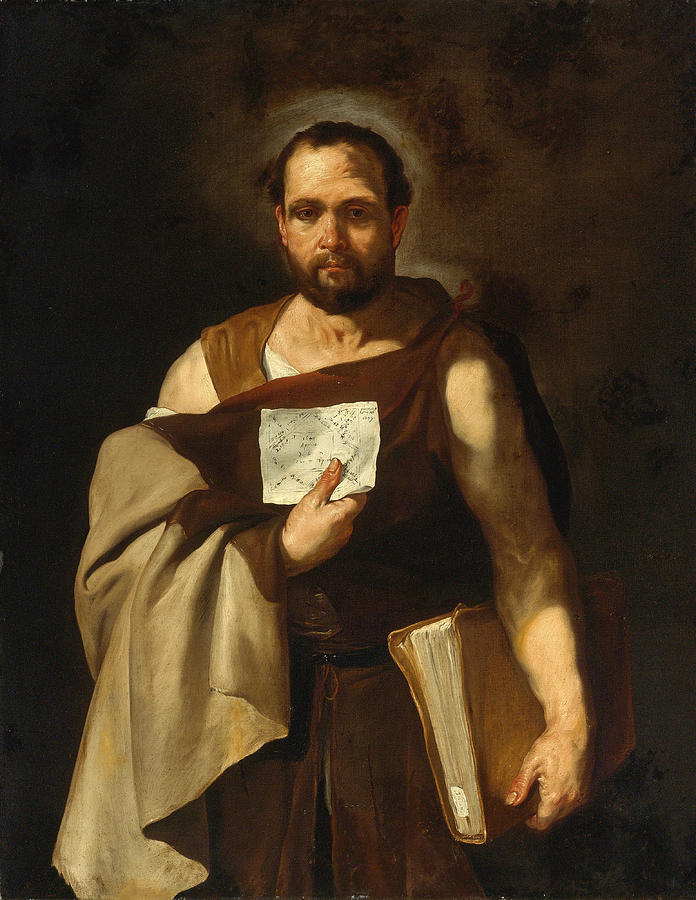This detailed painting depicts a man from a bygone era, possibly several centuries ago. He stands holding a large, thick, leather-bound brown book pressed against his left side, while his right hand clutches a piece of paper adorned with writings and sketches that resemble schematics. The man is clad in a flowing brown toga-like garment that drapes over his right shoulder and elbow, revealing a white undershirt beneath. His attire includes a brown dress-like outfit with a black belt and an asymmetric design: his left arm is sleeveless, showcasing muscular definition, while his right arm is covered by a voluminous white sleeve tied in a bow. The man, with short brown hair, a goatee, and a mustache, stands against a dark backdrop, which contrasts with the white light illuminating above his head. The intricate details of his attire and the focused expression on his face suggest he might be a scribe or scholar from his time.